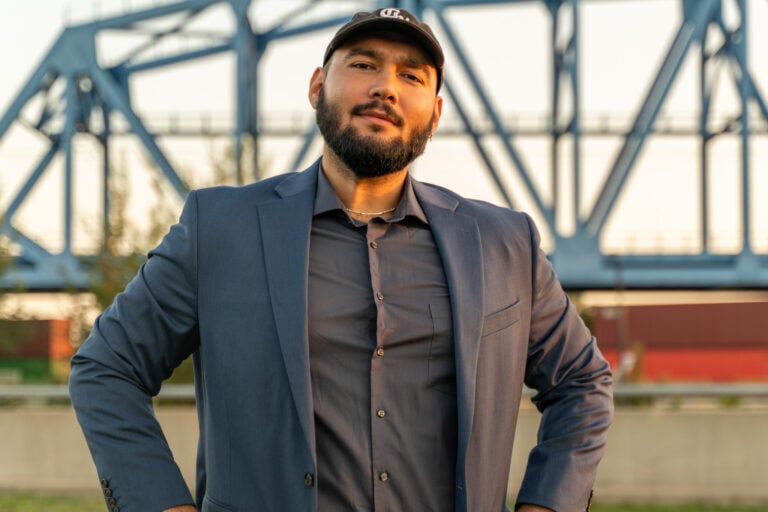The image depicts a man standing outdoors during what appears to be golden hour, indicated by the warm sunlight casting a glow from the left. The man has a dark complexion, with a full black beard and mustache, and is wearing a black baseball cap with white writing on it. He sports a relaxed, whimsical expression as he faces the camera. His attire includes a somewhat oversized gray sport jacket over a darker-gray button-up shirt that has the top button open, revealing a silver chain necklace. There's a hint of an earring in his left ear.

The backdrop features a striking blue steel structure, reminiscent of a small bridge or construction frame with a catwalk, and red buildings or objects at the base that resemble farmhouses or boxes. Additionally, there is visible greenery and a strip of asphalt or road accompanied by a gray guardrail, reinforcing the outdoor setting. The overall scene combines elements of rustic architecture and industrial design, adding depth to the man's poised yet casual stance.